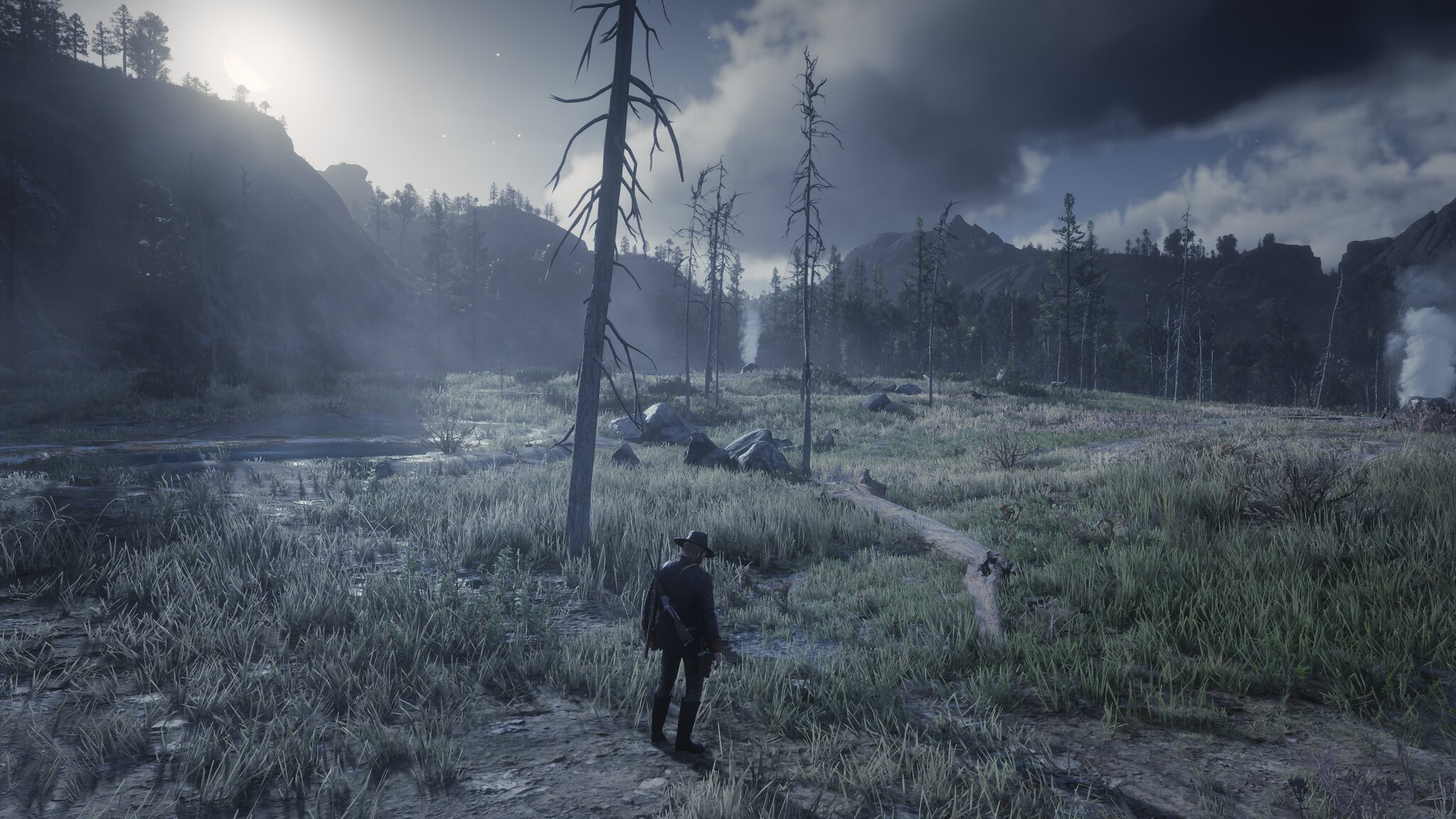In this detailed landscape shot from the video game Red Dead Redemption 2, we see the vast American wilderness as it might have appeared over a hundred years ago. The scene features a central character, viewed from a third-person perspective, who is wearing a cowboy hat and dark clothing, standing in a field that shows signs of previous fire damage. The man, small in the image, is facing away as he surveys the desolate terrain, with knee-high black boots, a dark jacket, and possibly a rifle slung over his shoulder along with other indistinct items, maybe a satchel.

The landscape is characterized by its rugged and barren features; dead, leafless trees—likely victims of fire—dot the field, along with scattered boulders and fallen trunks. The horizon showcases rolling hills that plateau to the left and distant mountain edges on both sides. The sky above is filled with a mix of large cloud formations and a dark, grayish hue, contributing to the somber atmosphere. Geysers and plumes of black smoke can be seen rising from several locations within the field, adding to the sense of desolation. The sun is either rising or setting, casting a low light and long shadows across the terrain, further emphasizing the dramatic and expansive vista.